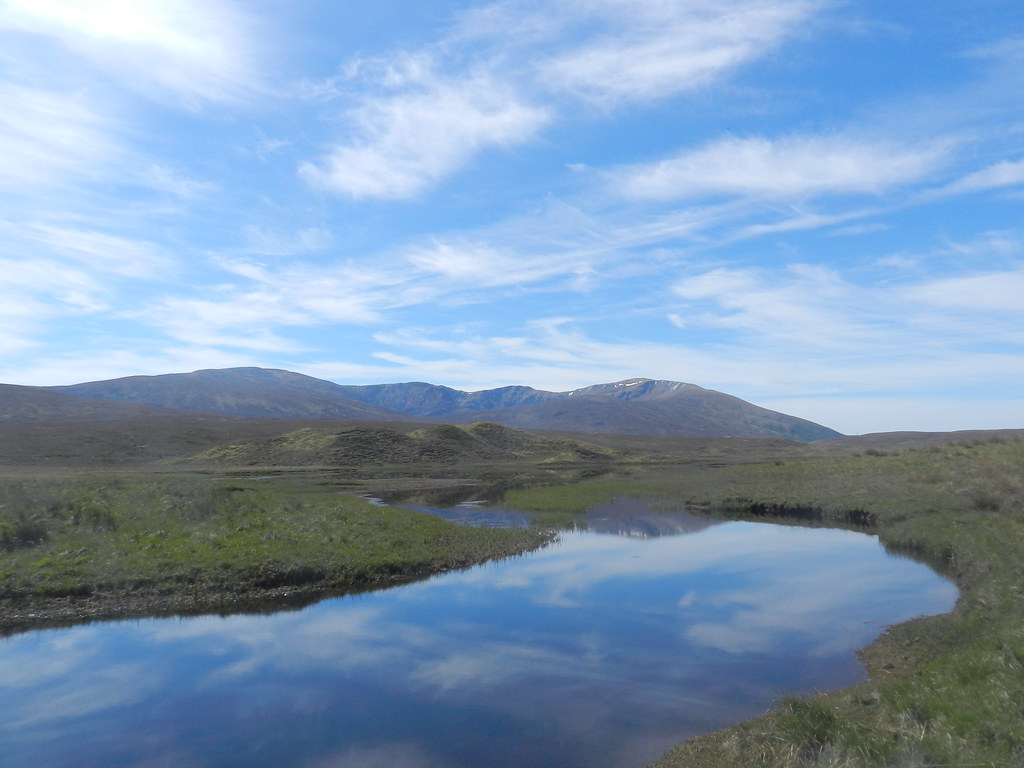A tranquil, winding body of water meanders through a grassy field, reflecting the blue sky and white, fluffy clouds above. The water’s surface is perfectly calm, without a single ripple, creating a mirror-like effect. It starts narrow in the center of the top of the image, curving gracefully left and right several times as it travels downward, gradually widening until it reaches the bottom corner. On either side of the water, the land is flat and covered with lush green grass, speckled with some weeds and patches of brown soil. In the distance, rolling green hills transition into larger, wavy mountains, which have a bluish tint. One particularly tall mountain in the center features streaks of white snow. The sky is a clear blue with a mix of sparse, fluffy clouds and a few cloud strips stretching across it.